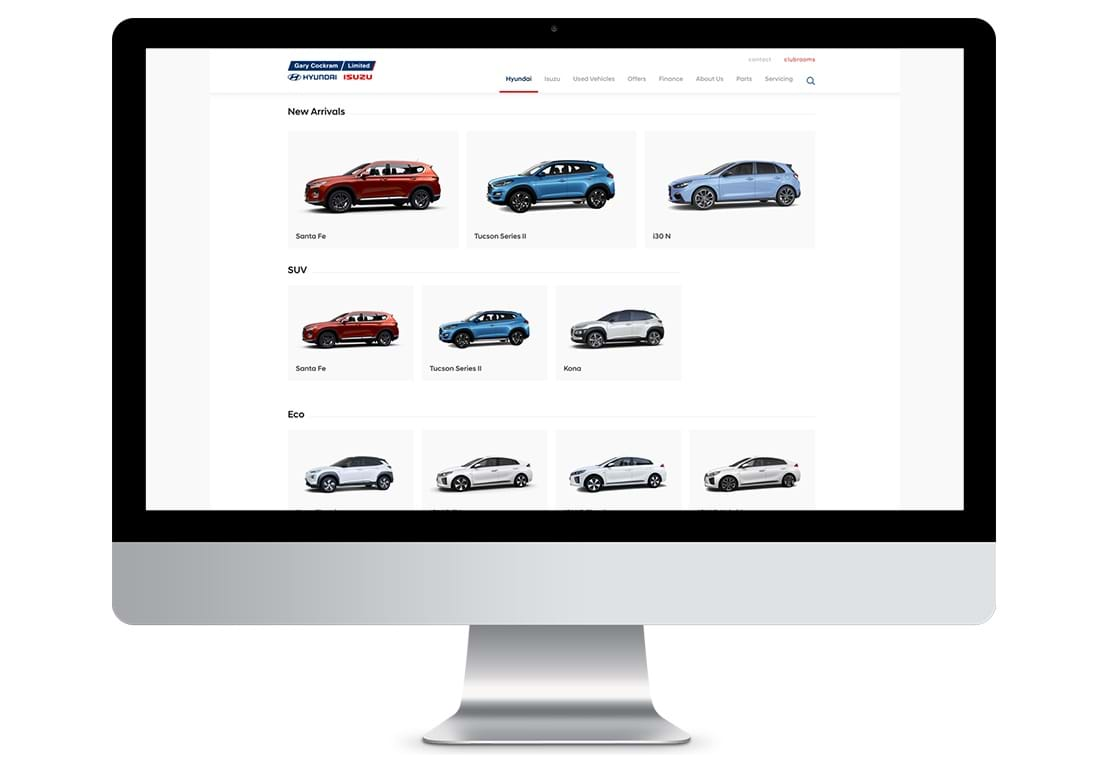An Apple desktop computer is prominently displayed, showcasing a website dedicated to vehicles, particularly highlighting Hyundai among other brands. The website interface features a series of menus at the top, which are quite small but legible. On the far-right side of the menu bar, a search icon is visible, allowing users to search for specific content within the site.

Beneath the main navigation, the site showcases high-resolution images of vehicles under the "New Arrivals" section, featuring orange, blue, and light blue cars. Further down, a distinctive section labeled "SUV" displays three vehicles in orange, blue, and white color schemes. Interestingly, the "Eco" section beneath it highlights four vehicles, all of which are white, making this stand out uniquely from the other sections.

The website's overall design features a white background with light grey tiles, placing emphasis on the vibrant images of the cars. This layout makes the vehicles the focal point of the page, ensuring they catch the viewer’s eye effortlessly. The contrast between the color-coded vehicles and the minimalist background provides a clean and visually appealing user experience.